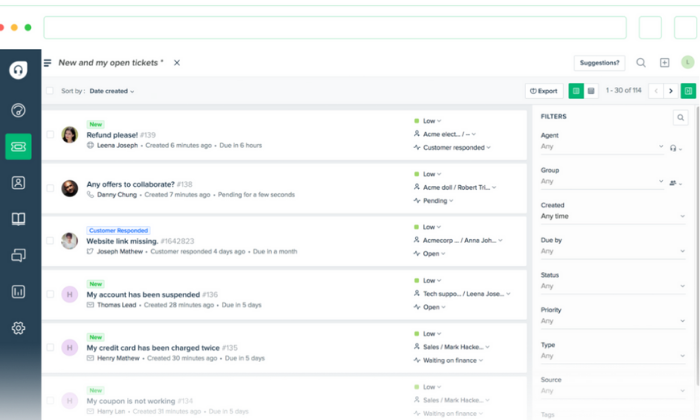This detailed website mock-up features a distinctive layout that includes various user interface elements. At the very top of the image, the browser bar is visible, distinguished by the characteristic red, yellow, and blue circle icons in the upper left corner. The border of the address bar is highlighted in green, accompanied by two additional green boxes positioned to its right, enhancing the appearance of a mock-up.

The left side of the webpage showcases a blue vertical menu bar adorned with several icons. At its summit is an icon that resembles a white teardrop paired with headphones. Below this, there is a circular icon followed by a green box icon, which contains another white symbol within it. Further down, the menu features icons in sequence: a small box with a person silhouette, an icon of a book, a chat icon, and a box flanked by two vertical lines with a smaller box in the center that reaches halfway up. A gear icon appears beneath these.

Adjacent to the blue menu bar, on the main section of the page, there is a prominently displayed heading: "New in My Open Tickets." Just below this heading, a gray box offers various options for management or sorting. Below this gray box, there are multiple entries, each formatted similarly: they showcase a person's profile picture on the left, a central message text, and additional options aligned to the right.

On the far right side of the webpage, a filter box labeled "Filters" is present. This feature provides multiple options to refine the items displayed on the website, allowing for a tailored user experience.